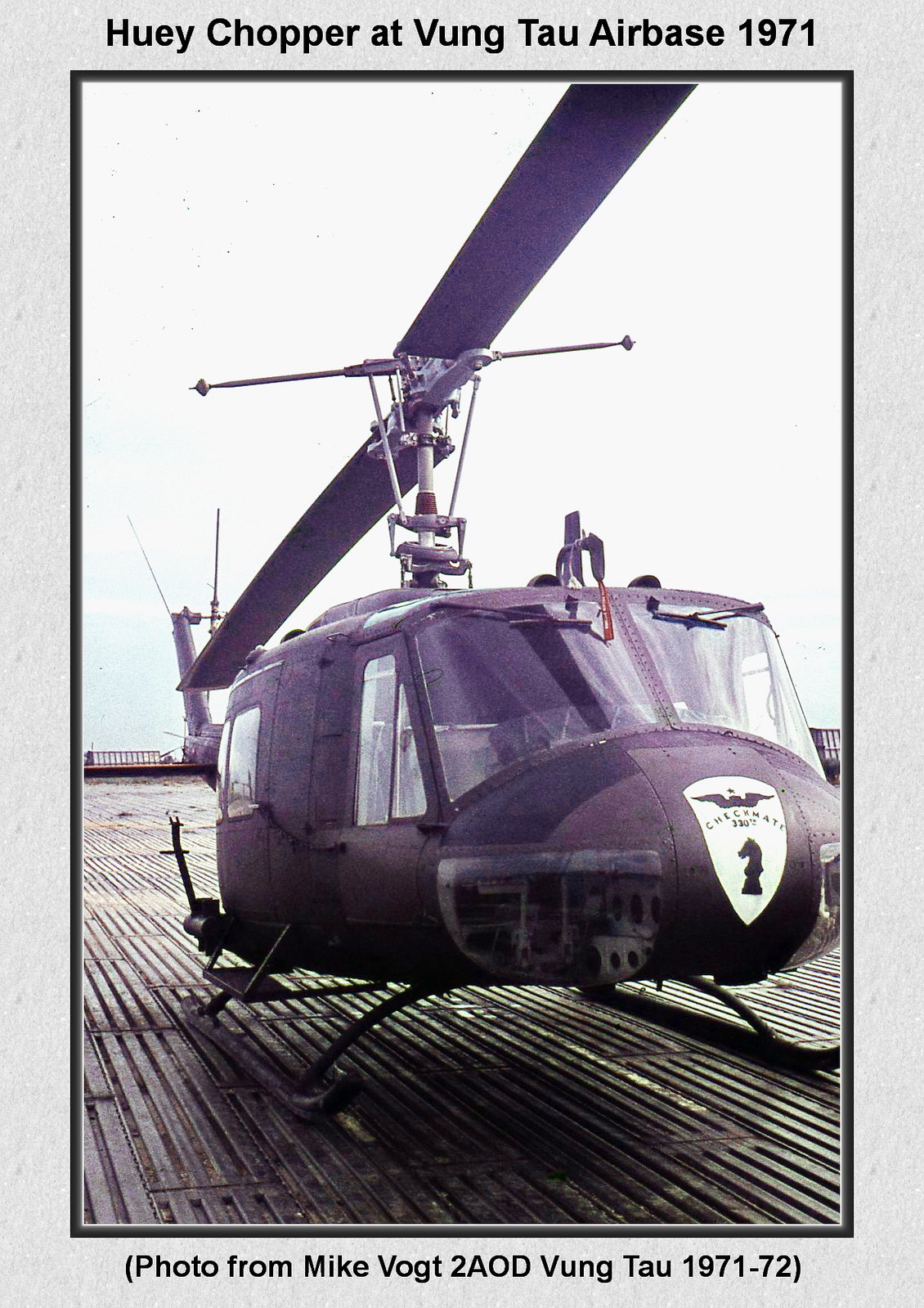The vertical photograph, framed by a narrow black outline, depicts a gray Huey helicopter at Vung Tau Air Base in 1971. The top caption in black letters reads, "Huey Chopper at Vung Tau Air Base, 1971." The helicopter is stationary, resting on what appears to be a metal grate surface outdoors, possibly a hangar deck or ground, with a cloudy white sky in the background. The helicopter rotor blades, aligned perpendicularly, stretch upward from the center towards the upper right corner of the image. The nose of the helicopter features a white shield logo, adorned with an eagle at the top and a knight chess piece at the bottom, with illegible text in between. The bottom caption, in black text on the white background, reads, "(photo from Mike Vogt to AOD Vung Tau 1971-72)."